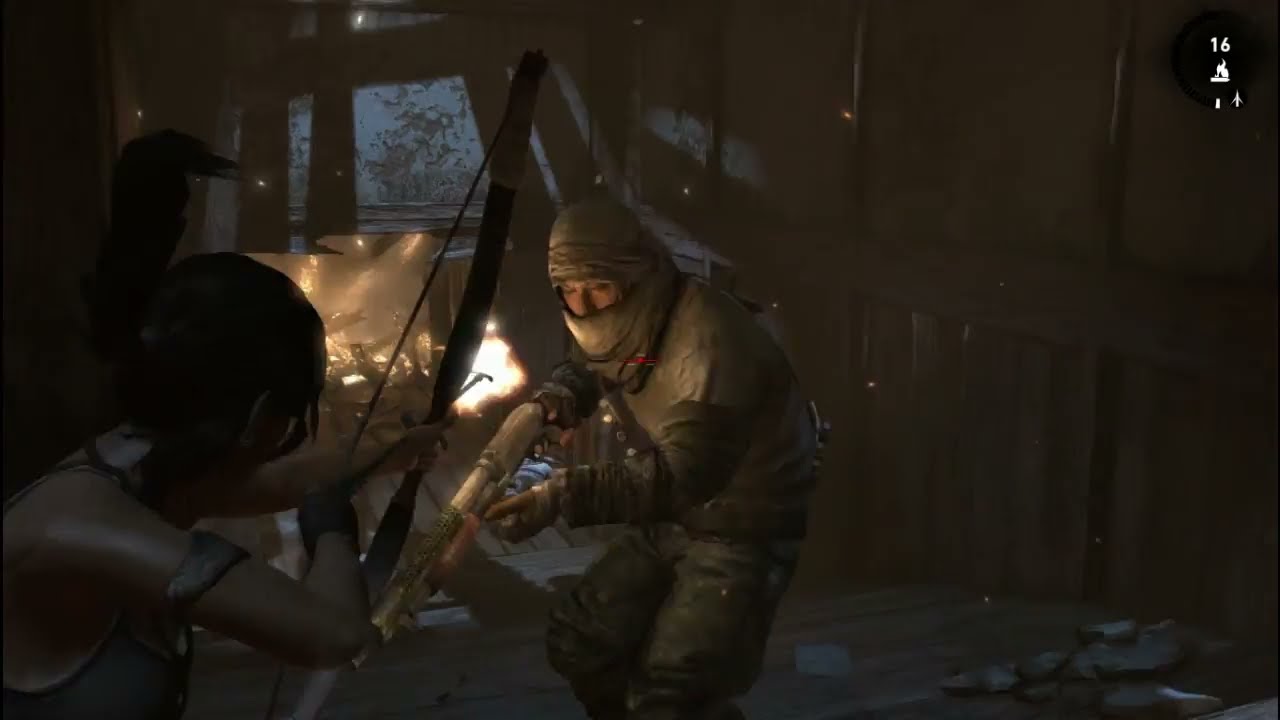The image, a still taken from a video game, depicts a tense standoff in a dimly lit, dilapidated shack. At the center is a soldier in full dark brown body armor and a headgear that obscures everything except their eyes and nose. The soldier is holding a gun, aimed towards the feet of an individual in the lower left foreground, who appears to be female. This individual has shoulder-length black hair—sometimes described as ponytail—clad in a strapless tank top, and is poised to release a flaming arrow from her bow aimed directly at the soldier. The scene takes place amid scattered wooden planks and debris on the floor, suggesting the shack's ruined state. The background, visible through broken walls, hints at a snowy or shadowy night-time environment. In the upper right corner of the image, a black circle with the number 16 and several icons are displayed, reinforcing the image's video game origin. A faint light from what seems to be a fire flickers in the lower left corner, adding to the scene's suspenseful atmosphere.